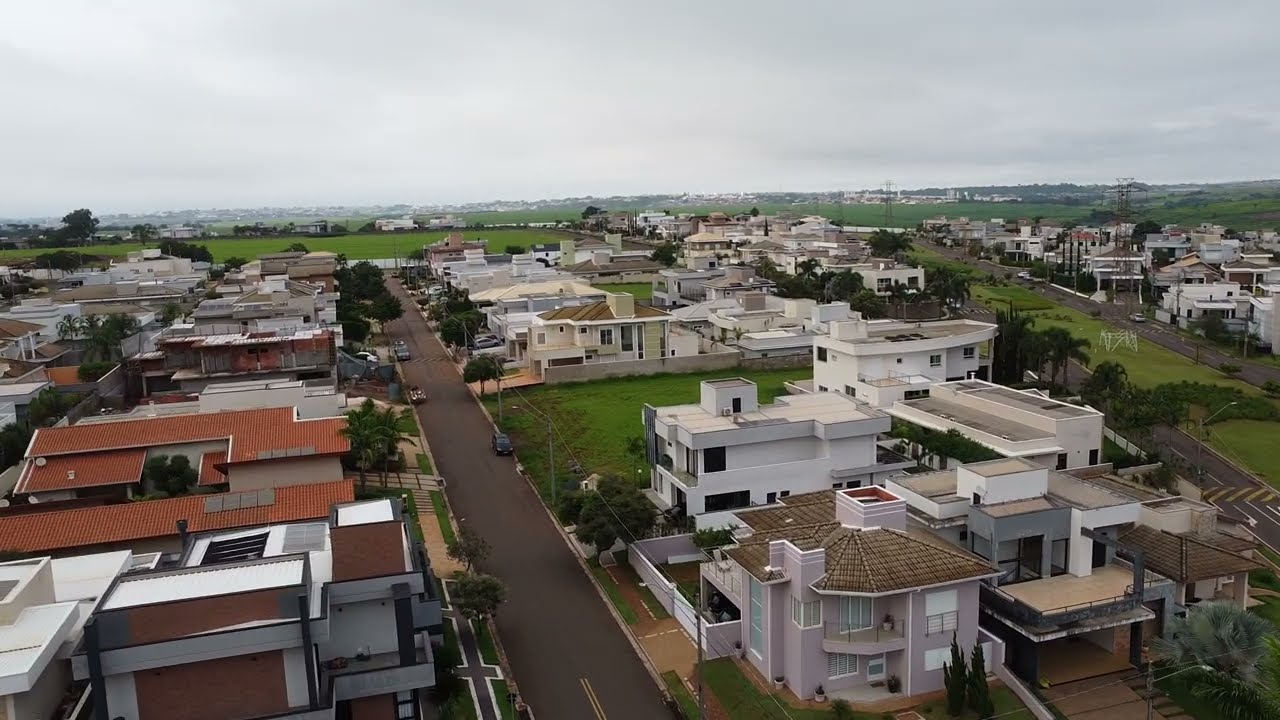The image depicts an upscale, modern neighborhood characterized by large, sleek, and blocky two-story houses predominantly painted white and light pink. This aerial view reveals a well-planned residential area with various buildings and gardens, interspersed with lush greenery and a multitude of trees, indicating a wet, non-desert climate. A road runs vertically from the bottom to mid-point of the image, with houses lined up on both sides. Cars can be seen driving on the roads, and there are additional roads branching out, dividing the residential blocks. Distinct architectural styles can be observed among the houses, including one prominent two-story stone house with an off-white facade and brown roof located in the lower right-hand corner. This house features a parking platform and is adjacent to a large circular building with a business-like appearance. In the background, there are rolling hills and a cloudy sky, adding to the picturesque setting. The presence of abundant grasslands and a small pond further enhances the neighborhood's serene ambiance.